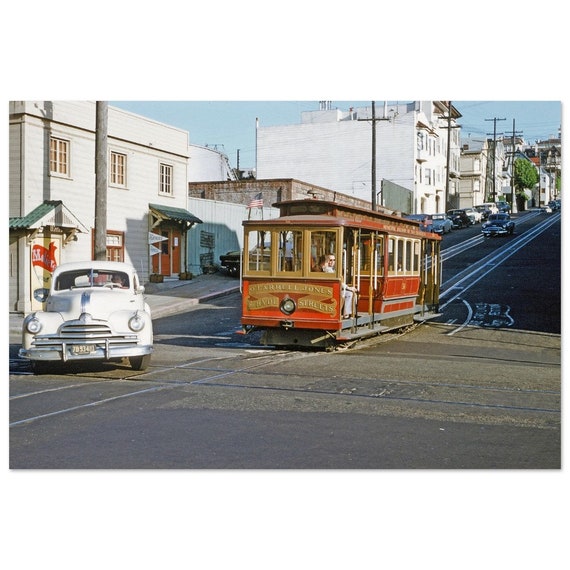This vintage photograph, likely from the 1950s, captures a quintessential scene of San Francisco. At the forefront, a white car resembling a Studebaker faces the viewer from the left side of the image. A classic red and gold trolley, characteristic of San Francisco cable cars, can be seen descending a slight hill toward the car. The trolley has a passenger dressed in light-colored attire, suggesting a pleasant weather day. The backdrop features a row of typical San Francisco stucco buildings, predominantly in various shades of white, none exceeding three or four stories in height. The scene is bathed in the golden light of late afternoon, with shadows cast along the right side. Cars are parked along the street, and telephone poles trace the path down the hill. The cloudless sky is a pale blue, emphasizing the bright, sunny atmosphere of this city snapshot. A single tree can be seen in the distance, punctuating the urban landscape of this bygone era.